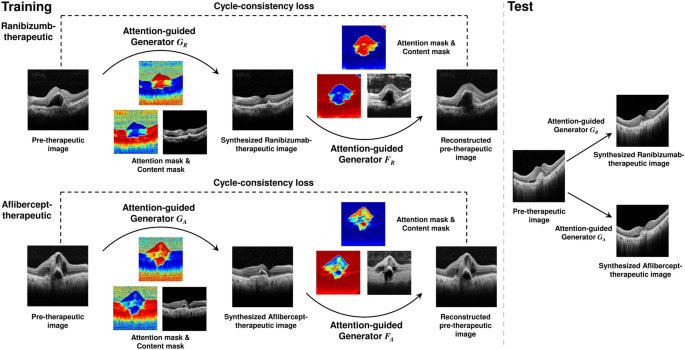The image presents a detailed medical chart illustrating the evaluation of therapeutic effects. The chart comprises several sections including training and test phases, showcasing a variety of diagnostic images. On the left, beneath the label "Ranibizumbab Therapeutic," a flow diagram featuring a series of boxes contains photographs of thermal and x-ray images, used to determine the efficacy of the therapy. Highlighted terms include "Attention Guided Generator," "Attention Mask," and "Content Mask." The central part of the chart details "Cycle Consistency Loss for Afibercept Therapeutic" with associated images.

On the right side, labeled "Test," the chart contrasts pre-therapeutic and synthesized therapeutic images, featuring both black-and-white x-ray images and color-coded thermal images employing red, green, and blue hues. The images are organized in a comparative manner to assess the therapeutic outcomes. This comprehensive chart is an amalgamation of several diagnostic techniques aimed at training and gauging the effectiveness of different therapeutic interventions using advanced medical imaging technology.